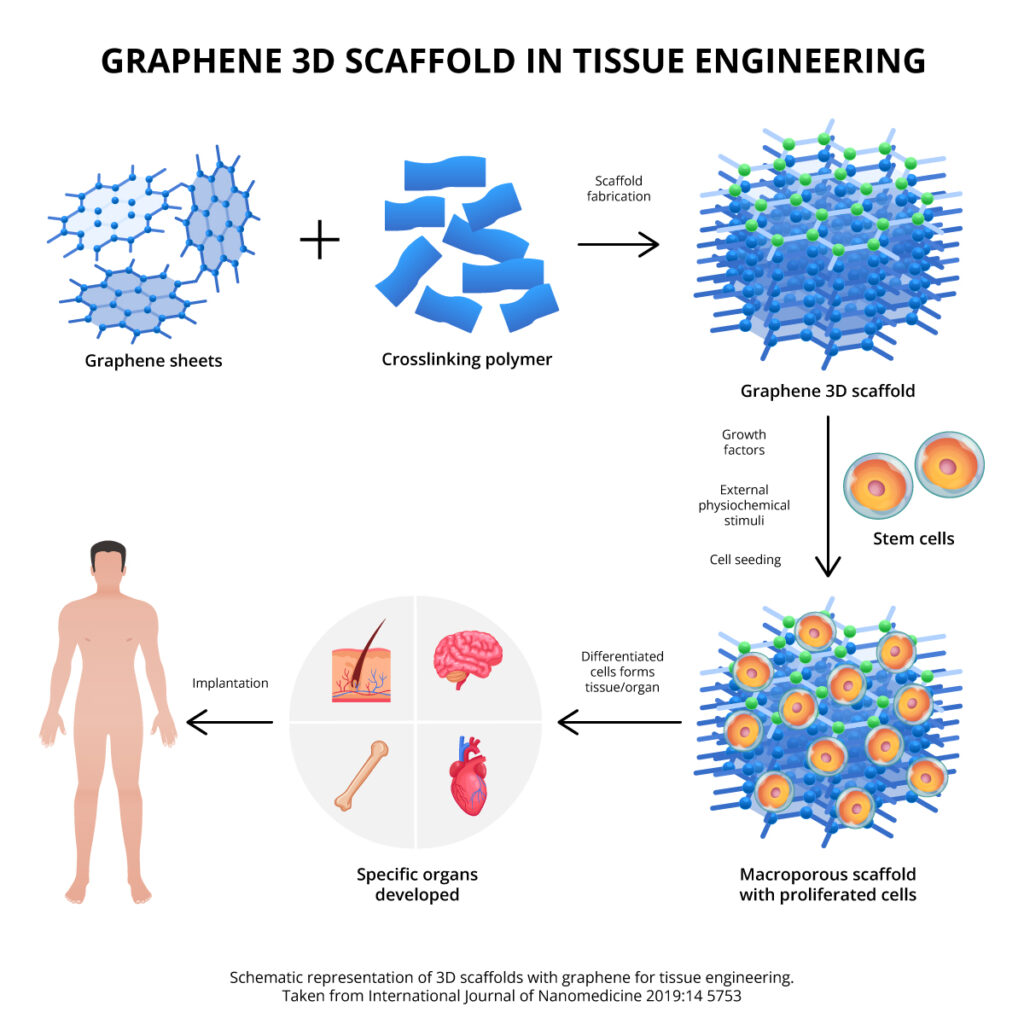The image is a comprehensive diagram titled "Graphene 3D Scaffold in Tissue Engineering" on a plain white background. It starts with an illustration of graphene sheets combined with a cross-linking polymer, leading to the scaffold fabrication process, resulting in a Graphene 3D Scaffold. Stem cells are then introduced alongside growth factors, external physiochemical stimuli, and cell seeding. This process facilitates cell proliferation within a macroporous scaffold. The ensuing stage depicts the differentiation of cells into various tissues and organs, including hair, brain, bone, and heart. Finally, the diagram illustrates the implantation of these developed tissues/organs into a human body. Additionally, the diagram is noted to be a graphic representation of 3D scaffolds with graphene for tissue engineering, sourced from the International Journal of Nanomedicine, 2019-14-5753.